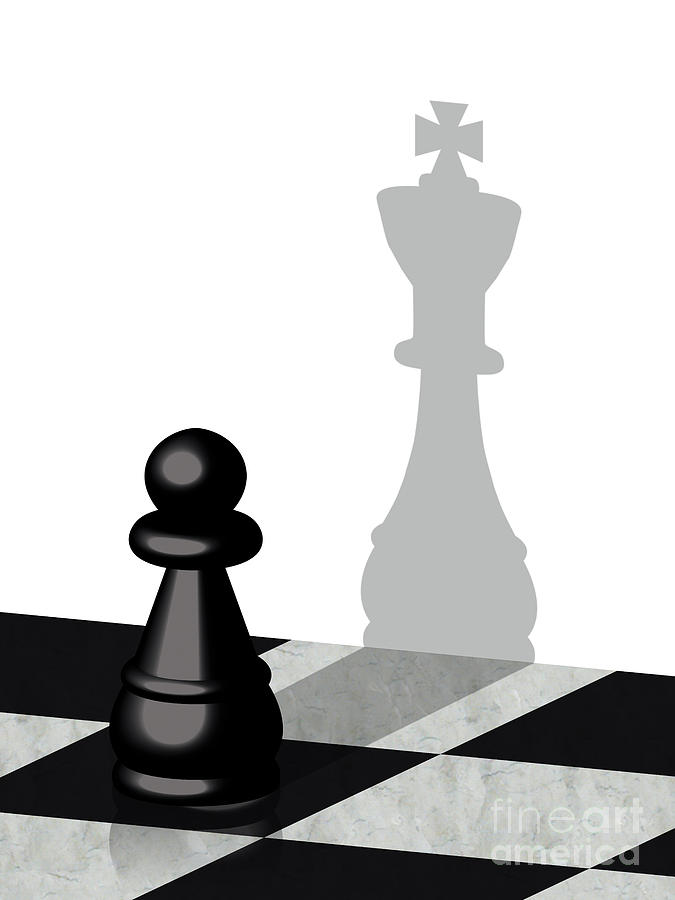This artistic black-and-white photograph captures a fascinating scene on a chessboard. A small black pawn, with a round head and narrow body, rests on a black square. Though dwarfed in stature, the pawn casts an intriguing shadow against a stark white background. The shadow is not of the pawn itself, but of a much larger king chess piece, complete with a cross-topped crown and elongated body. The juxtaposition highlights a dramatic transformation from the humble pawn to the majestic king within the same frame. In the bottom right corner of the composition, the watermark of Fine Art America, semi-transparent, subtly blends into the monochromatic theme. The partially visible black-and-white checkered board adds depth, enhancing the overall minimalist yet powerful visual narrative.